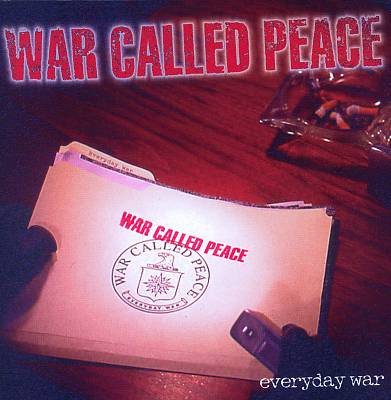In this image, a dimly lit scene unfolds upon a wooden desk. Centered on the desk is a thick, manila folder brimming with papers, gripped by two hands clad in black gloves—one on the left, merely the thumb visible, and the other on the right, potentially holding a stapler. Stamped prominently in red across the top of the image, the front of the folder, and within an official-looking round seal, are the ominous words, "War Called Peace." The round seal showcases an eagle's head, facing left and clutching what appears to be a shield. Above the folder and towards the top right corner of the image, a glass ashtray holds three smoldering cigarette butts, contributing to the clandestine atmosphere suggestive of a detective or undercover operation.